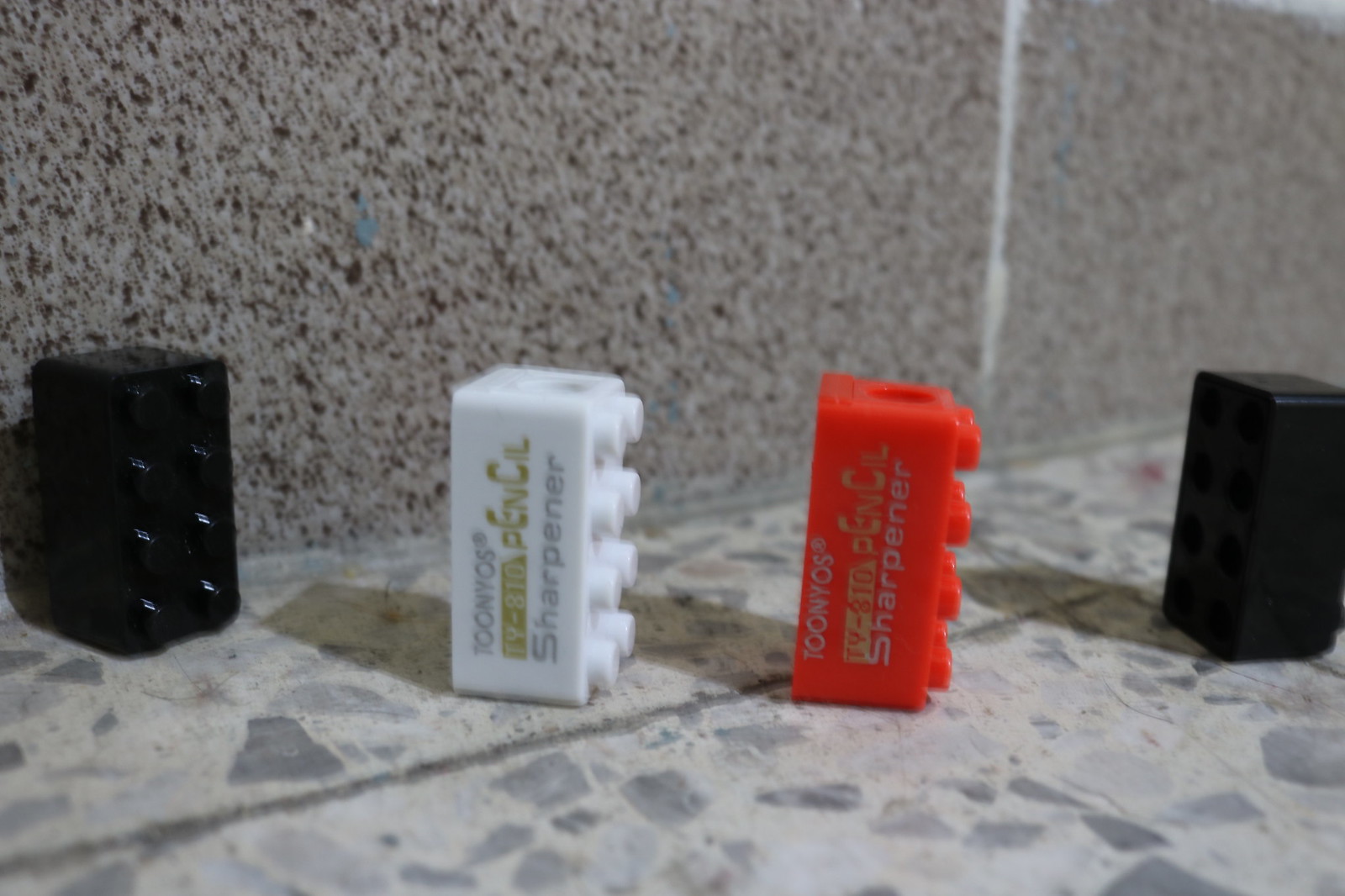In this detailed close-up photograph taken from a low angle, the focus is on four small, upright Lego-shaped plastic objects, resembling motors from a Lego clone set. These objects are situated on a rough, stone-like surface composed of various irregularly shaped stones mixed into asphalt-like material. The surface features a mixture of light gray, dark gray, and tan rocks, reminiscent of a beach lined with pebbles.

The objects are positioned against a background of light brown and gray tiled wall with white grout interspersed with chocolate brown and black specks. The tiles create a marble-like effect, enhancing the visual texture of the setting.

Each of the four Lego-like pieces has a rectangular shape with circles on the back, designed for fitting connection pieces, similar to Lego bricks. The pieces, which are pencil sharpeners, display the words “sharpener” and “pencil sharpener” on them. The first piece on the left is solid black. Next comes a white piece with the writing “Tunios Pencil Sharpener” on it. The third piece is red with similar labeling, and the final piece on the right is another solid black piece facing away from the camera.